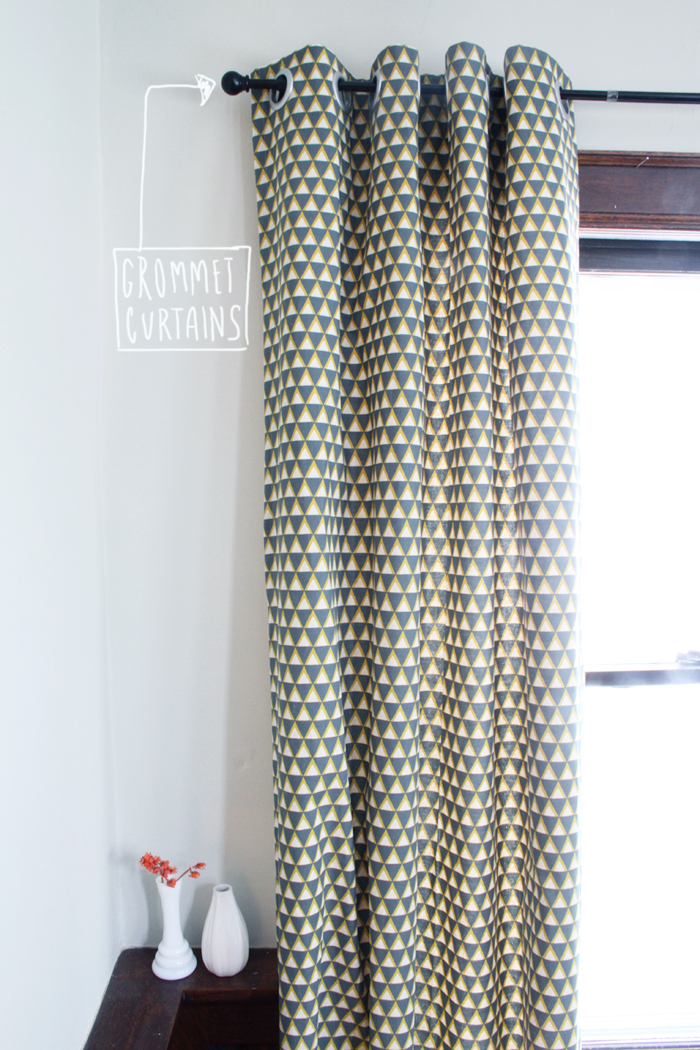This detailed photograph, in portrait orientation, features a single curtain panel hanging from a narrow black rod with a ball finial, positioned about a quarter of the way down from the top of the image. The curtain, described as either dark blue, dark gray, green, or gray, displays a repeated pattern of triangles, some with yellow outlines or pyramids. The curtain covers a tall window with a black frame and a brown wood trim. Light streams through the window, obscuring the view outside. 

At the bottom left corner of the image, a dark wooden table or ledge holds two white ceramic vases, one of which contains a few red or orange flowers. A prominent feature near the top of the image is a white arrow pointing towards the curtain rod from a white-outlined box, with the text “Grommet Curtains” written in white letters. The wall behind the curtain is described as either gray or white. The style of the image is photographic representationalism realism with added textual elements.